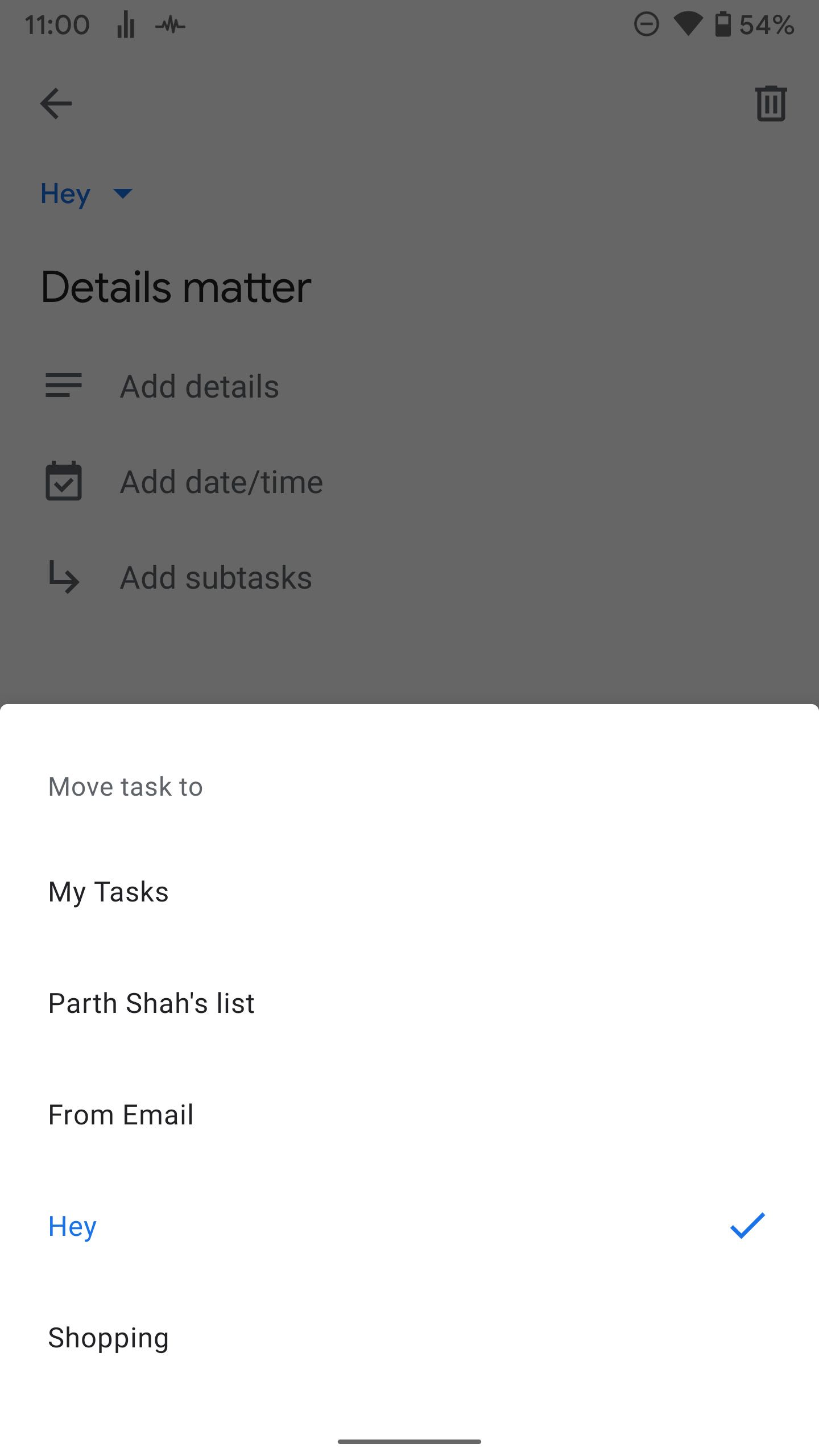The screenshot captures the interface of a Lists app on a mobile phone displayed in landscape mode. The upper part of the screen features a semi-transparent black overlay. At the bottom, a white pop-up box obscures part of the background.

Inside the pop-up box, a vertical list titled "Move Task To" displays several options: "My Tasks," "Parth Shah's List," "From Email," "Hay," and "Shopping." The option "Hay" is selected, indicated by a small blue checkmark to the right and the word itself is highlighted in blue.

In the background of the screenshot, at the top left corner, there is a small drop-down box also showing "Hay" selected in a light blue color. Directly below it, the bold text "Details Matter" is prominently displayed. Beneath this title, three options are listed: "Add Details," "Add Date and Time," and "Add Subtasks."

In the top-right corner of the screenshot, a trash can icon is visible, suggesting an option to delete items. On the top-left side, there's a back arrow, providing navigation to the previous screen.